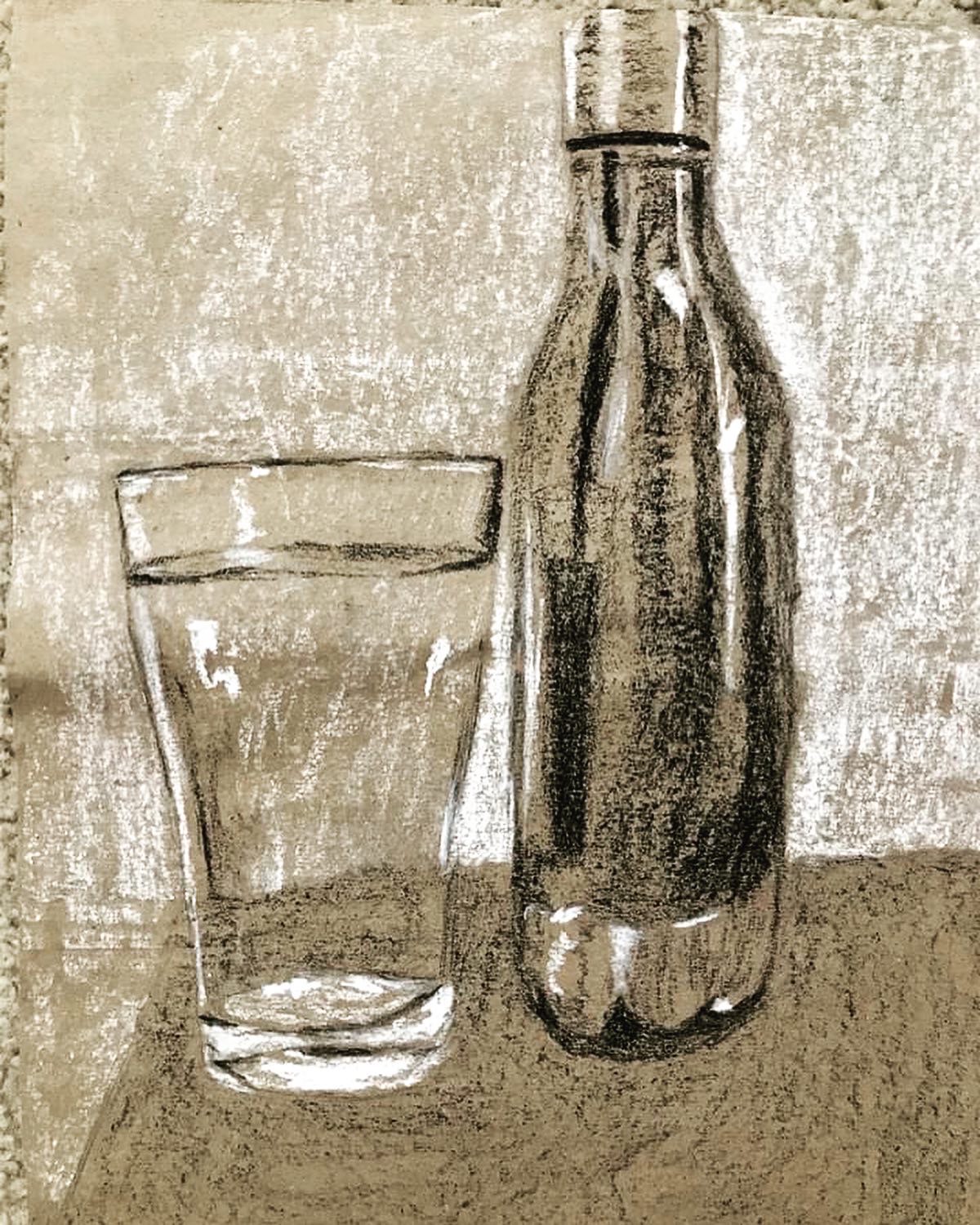The image depicts a scene with a predominantly brown background, which also extends to the bottom of the frame. The brown base is interspersed with black markings. Scattered throughout the brown background are subtle white marks that add contrast to the scene. In the foreground, there are two glass jars positioned side by side. The jar on the left is filled with a liquid that captures ambient reflections, giving it a glossy appearance. The jar on the right is capped with a silver lid, which is notably reflective. This jar features a combination of white reflective highlights along its sides and black markings in the middle, suggesting residues or liquid marks. The overall composition highlights the textures and reflective qualities of the jars against the richly colored background.